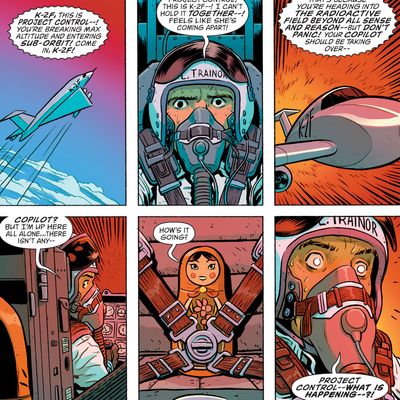This vibrant and colorful six-panel comic strip vividly illustrates a high-stakes scenario involving a jet aircraft and its pilot. In the first frame, a jet aircraft breaks through the sky, accompanied by a communication from Project Control: "K2F, this is Project Control. You're breaking maximum altitude and entering suborbit. Come in, K2F." The second frame zooms in on the pilot's face, who responds, "This is K2F. I can't hold it together. Feels like she's coming apart." The third frame returns to the jet's exterior as Project Control advises, "You're heading into the radioactive field beyond all sense and reason, but don't panic. Your co-pilot should be taking over."

The tension escalates in the fourth frame when the pilot realizes his dire situation: "Co-pilot? But I'm up here all alone. There isn't any..." Suddenly, in the fifth frame, the comic humorously reveals a Matryoshka doll, a Russian nesting doll, strapped into the co-pilot's seat, casually asking, "How's it going?" In the final frame, the pilot, now visibly panicked, exclaims, "Project Control, what is happening?" This blend of suspense and surreal humor effectively captures the chaotic and absurd nature of the pilot's predicament.